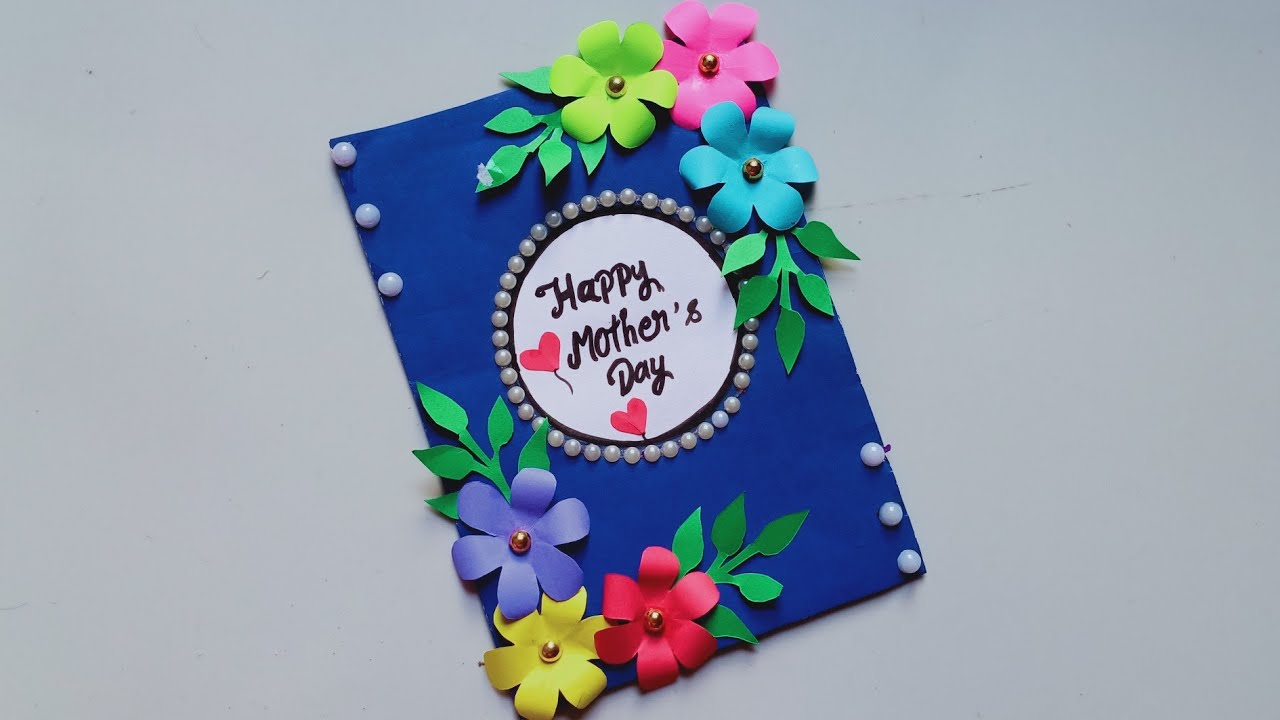This image showcases a beautifully crafted handmade Mother's Day card set against a light gray background, displayed on a light blue table. The card itself is made from dark blue crepe paper, folded to form a greeting card. The centerpiece of the card is a large, white circular cutout, bordered with glued white pearls. Within the circle, "Happy Mother's Day" is elegantly scripted in black cursive, accompanied by two red heart balloons to the left.

In the upper right corner, there is a cluster of three 3D paper flowers in green, pink, and blue, each centered with a gold pearl. Greenery accents extend from this flower arrangement to the left and bottom. Mirroring this arrangement, the lower left corner features a similar cluster with purple, yellow, and red flowers, also centered with gold pearls, and greenery extending to the top and right.

Additional decorative elements include three pearls arranged vertically in the upper left corner and three in the lower right corner of the card. The card is tilted approximately 20 degrees to the left, highlighting the intricate details and the care put into its creation.